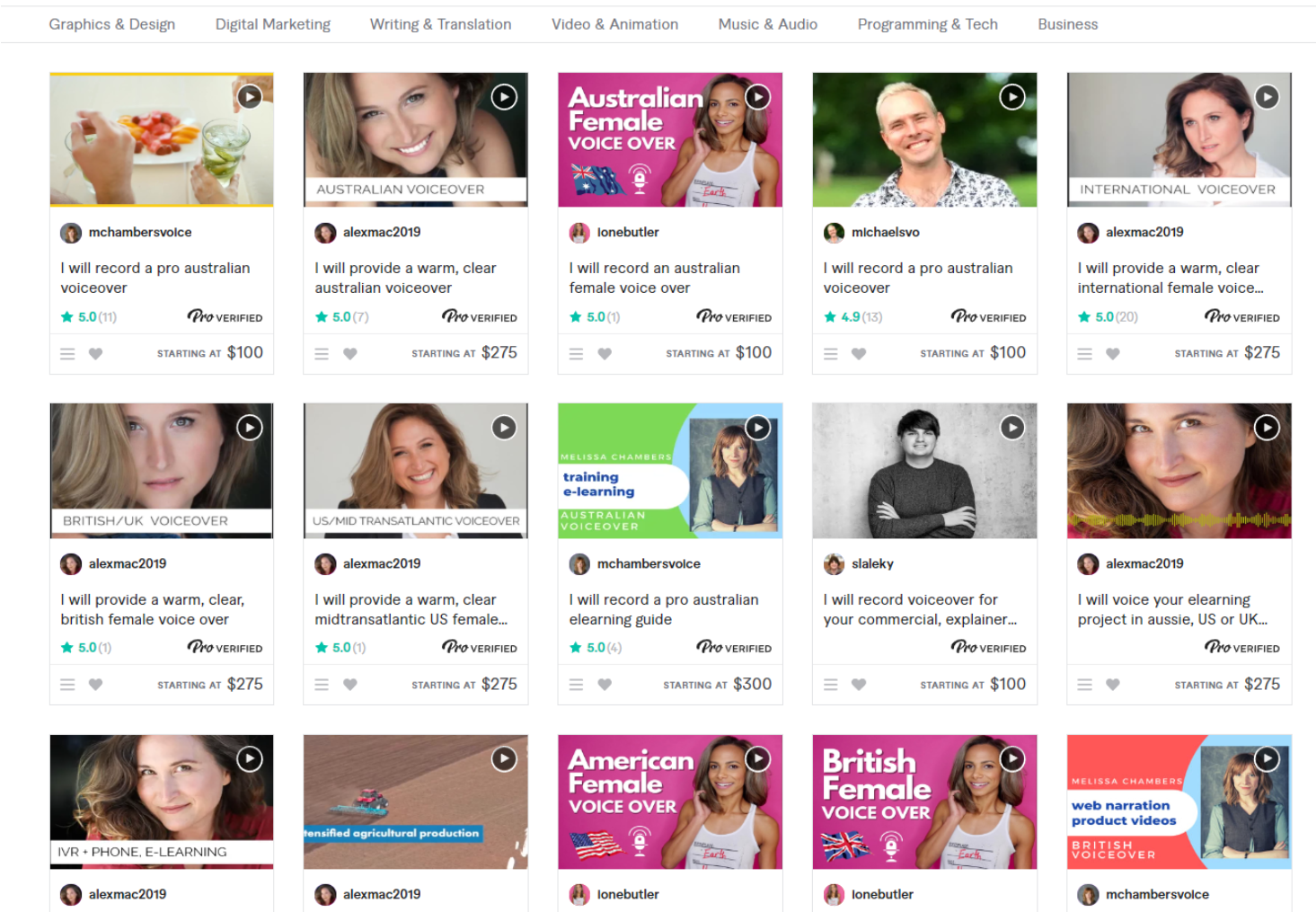The image depicts a webpage showcasing a variety of freelance service listings, specifically focusing on voiceover talent. The layout consists of three rows, each containing five listings, bringing the total to fifteen visible options. The majority of the listings feature a cheerful woman, though some include men as well. The services are organized under several sections: Graphics & Design, Digital Marketing, Writing & Translation, and Video. This suggests that the website is a platform for learning and skill acquisition, similar to sites like LinkedIn Learning (formerly Lynda).

Upon closer inspection, it becomes clear that the site is a freelance marketplace. Each listing includes a service description, starting price, and user rating. For instance, one listing offers "Australian voiceover" services, promising a warm and clear voiceover starting at $275, and boasts a five-star rating based on seven reviews. 

A frequently featured provider, identified as Alex Mac 2019, appears in several listings. Another provider, Michael SVO, offers professional Australian voiceovers. It appears the search query used might have been specifically for Australian voiceover artists, given the repeated emphasis on this category.

In summary, the webpage is a detailed display of various freelance voiceover services, prominently featuring Australian voiceover artists and showcasing vital information such as service descriptions, starting prices, and user ratings.